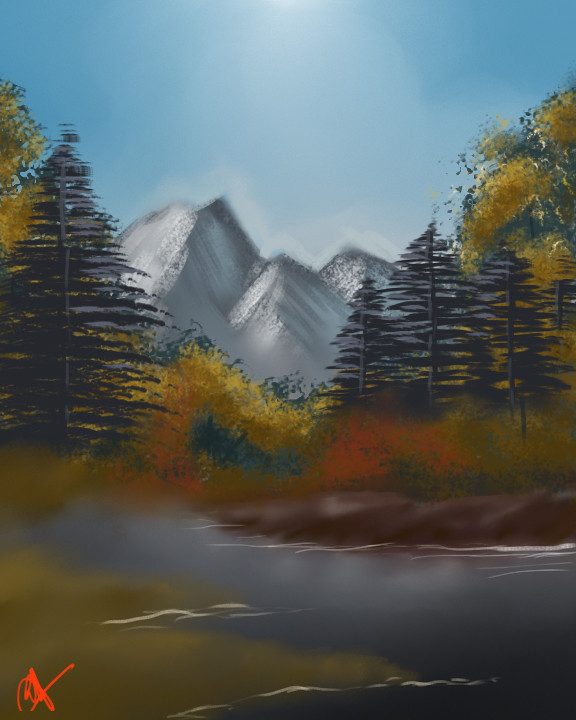This detailed painting, possibly rendered with oils, presents a captivating autumnal landscape set in a rectangular, upright frame. The scene is dominated by three tall, triangular mountain peaks, dusted with a light skiff of snow that subtly merges into the blue sky above. On either side of the mountains, a mix of green pine trees and deciduous trees with yellow and orange leaves indicates the fall season. At the foot of the mountains, the foreground is adorned with yellowish bushes and orangish grass, blending into a brown, earthy riverbank. A small pool of water, dark blue and slightly foggy, mimics a serene lake or stream, complete with white highlights that suggest flowing water. The very bottom of the painting reveals a rocky and grassy area, with the artist's signature, resembling a red scribbled X, in the lower left-hand corner. This artwork beautifully captures the essence of a tranquil autumn day in nature.